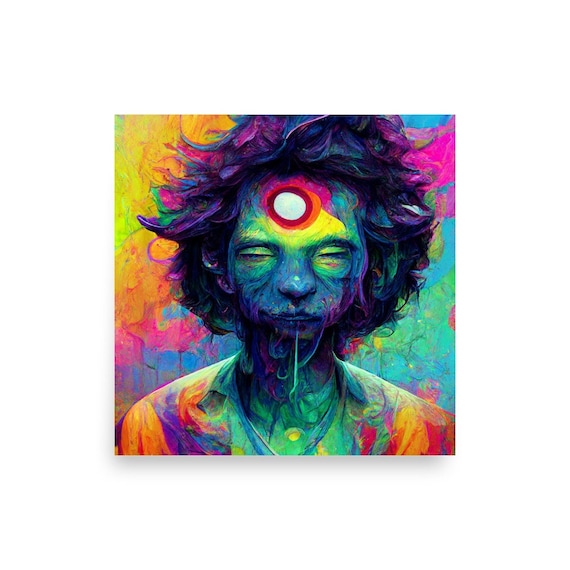The image is a highly detailed, abstract, and modern portrait of a man with a psychedelic, kaleidoscopic aesthetic. His eyes are closed, and his broad face, featuring a broad nose and thin lips, suggests a serene expression. His hair is medium-length, curly, and wild, with hues of purple and blue. The man has facial hair, including a thin beard starting from his bottom lip. A striking feature is the hole in his forehead, a white center encircled by layers of deep red, orange, and pink. The colors of his face transition between green and blue, while his neck blends into blue and green shades. He is wearing a collared shirt painted in green, purple, and orange tones. In the background, the top left corner is dominated by yellow and orange, the top right by blues, greens, and pinks, while the bottom corners display a mix of green, pink, blue, orange, and purple. This portrait captures the essence of a vibrant and dynamic modern artwork.